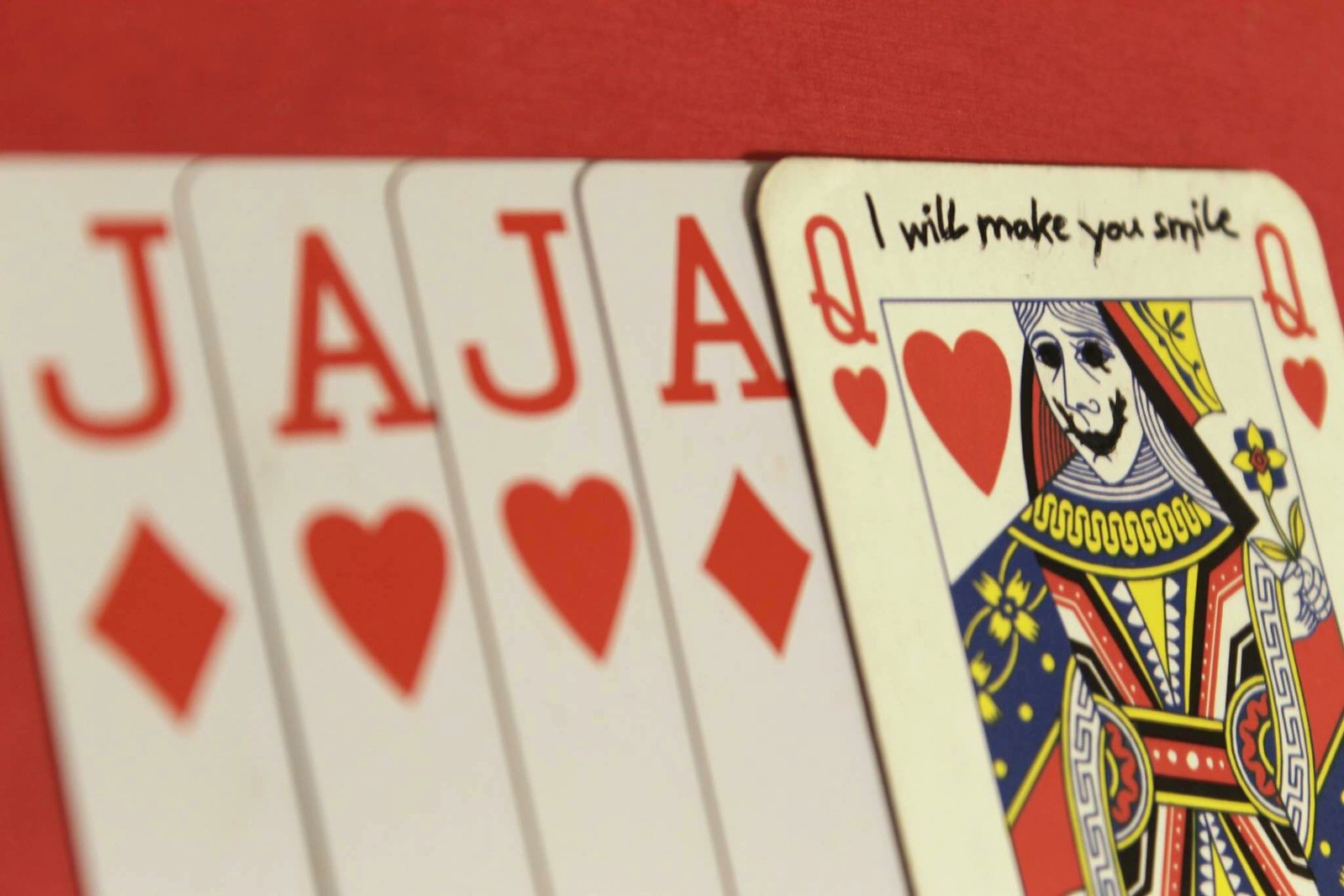On a vibrant red background, five striking playing cards neatly align in a horizontal row. These cards, all part of the red suit, alternate between diamonds and hearts, arranged in the following order: Jack, Ace, Jack, Ace, and Queen. The cards are partially overlapped, revealing only the suit icons and the corner ranks on narrow vertical strips to the left. The rightmost card, however, is fully visible, showing the Queen of Hearts in her entirety. 

Upon closer inspection, a message written in fine ballpoint pen or marker adorns the Queen of Hearts card. Just above the card's emblem, nestled between the two 'Q's, the note reads: "I will make you smile." Additionally, the face of the Queen is altered with a large, eerie grin drawn over her serene expression, with sharp, spike-like lines extending from its edges. Her eyes are filled in with black, also extending into spiky protrusions, creating a haunting visage that strikingly contrasts with the otherwise regal imagery.